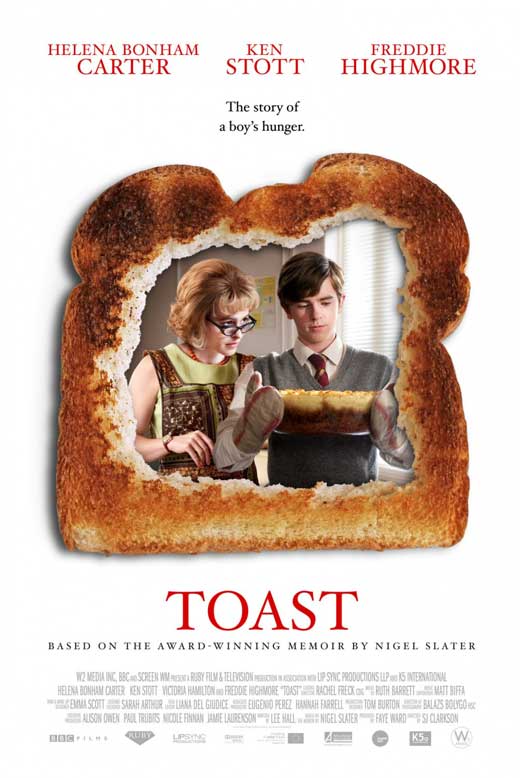**Caption for Movie Poster:**

The poster features a simple white background. Across the top left corner, the name "Helen Bonham Carter" is prominently displayed in red lettering. Just below her name, equally in red, is "Ken Stott," and to the top right, "Freddie Highmore."

In the center of the poster, slightly below Ken Stott's name, is a smaller, black text that reads, "The story of a boy's hunger period." Directly beneath this text is an image of a piece of toast, charred around the edges with a section peeled out in the middle. Inside this peeled-out section is a photograph of a woman and a boy standing inside a room.

The woman is positioned on the left side of the image, facing the camera with her head tilted slightly downwards to the right. She has short, reddish-blonde hair, wears black glasses, and is dressed in a green shirt over which she dons a brown apron. Her demeanor suggests a blend of sternness and affection.

Standing to her right is the younger man, who has short, brown hair and is focused intently on a dish in his hands. He wears a neatly tied red tie, a gray vest, and long-sleeved white shirt, complemented by white oven mitts holding a casserole dish. The backdrop behind them is a plain white wall, with a window on the right side covered by white blinds.

Below the toast, in bold red letters, the title "Toast" is prominently displayed. Beneath the title, in smaller black text, it reads, "Based on the award-winning memoir by Nigel Slater." Finally, all the credits for the various contributors to the movie are listed neatly at the bottom of the poster.